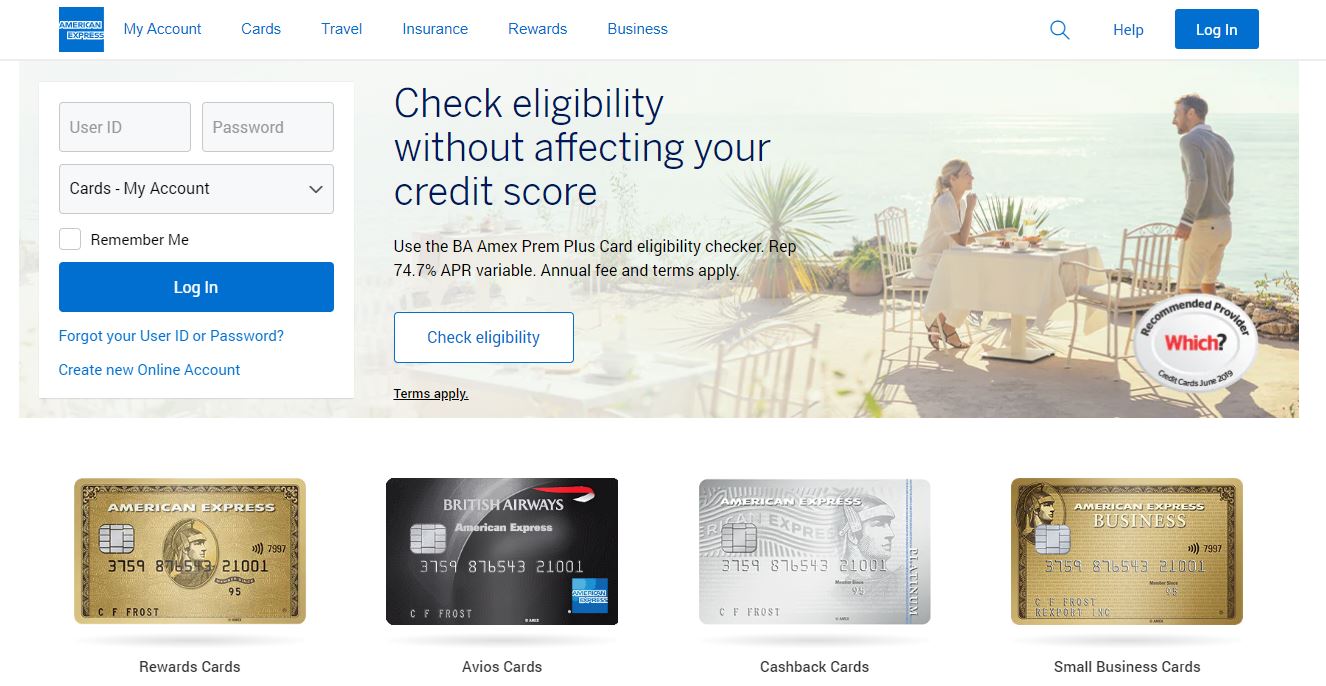The image depicts an American Express website with a predominantly white background. In the top left corner, a blue square bearing the white text "American Express" stands out. The top navigation bar is adorned with blue text labels for various sections of the website: Buy Account, Cards, Travel, Insurance, Rewards, and Business. 

On the top right, there's a prominent blue "Log In" button, flanked to its left by a "Help" link and a "Search" button.

Beneath the main content are four distinctively colored cards arranged from left to right: gold, black, grey, and another gold card. Below these cards, black text labels categorize them as Rewards Cards, AVOs Cards, Cash Back Cards, and Small Business Cards. Notably, the black card is inscribed with "British Airways" and "American Express," while the others simply read "American Express" in white text.

Dominating the center of the page is a large banner featuring a luxurious scene: a man and a woman dine at a table overlooking a vast and tranquil body of water. The right side of the banner highlights this serene setting, which gently fades into a plain background on the left side. Here, a white rectangular form displays input fields for "User ID," "Password," and "Cards by Account," alongside a blue "Log In" button. 

Prominently placed at the center of the banner, bold text invites users to "Check Eligibility Without Affecting Your Credit Score" using the AMEX Credit Card Eligibility Checker, accompanied by a "Check Eligibility" button. The banner also boasts a white circular emblem at the bottom right, proudly announcing "Recommended Provider, Which Credit Card Since 2019."